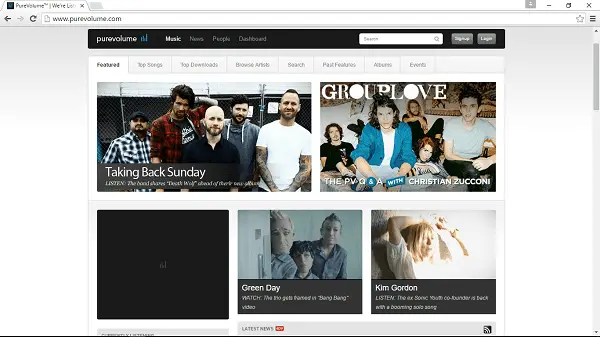The image is a small, somewhat unclear screenshot of a computer screen displaying a webpage from a music website called PureVolume.com. The homepage features various artists. At the top left, there's an image of the band Taking Back Sunday, comprising five members. Adjacent to this, on the right, is a photo of the band Grouplove, which also has five members. Below these images, additional bands are listed. An advertisement space is present but appears blocked, showing only a large black square with a small gray icon in the center. Next to the blocked advertisement, there's a section for the band Green Day, a trio. In the bottom right corner, the screenshot features Kim Gordon, recognized as a music recording artist and likely a singer.